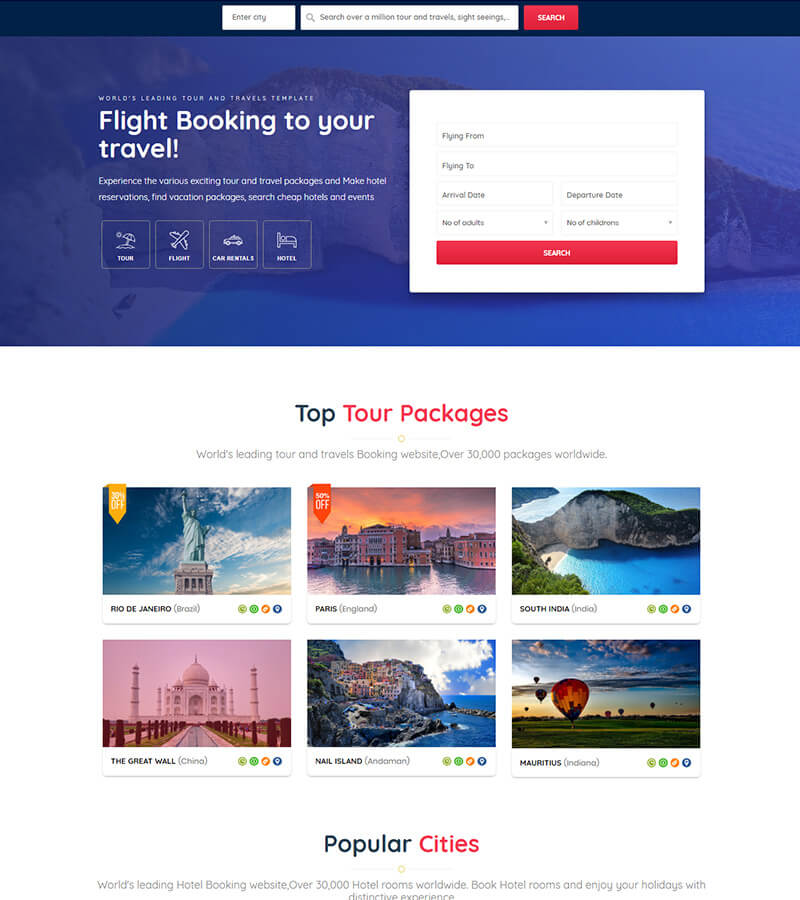The image depicts the main page of a travel agency's website, characterized by its distinctive purple background. Dominating the page is a bold headline proclaiming "World's Leading Tour," followed by a subheading, "Flight Booking to Your Travel," both slightly difficult to read due to size.

Below this header, four small interactive dialog boxes are lined up, designed for users to engage with. The topmost section of the page features a prominent search function, enabling users to specify their destination. Adjacent to this search bar are additional fields where users can input details such as "Flying From," "Flying To," "Arrival Date," and "Departure Date." These fields facilitate the search for the best available flight options.

Beneath the flight search section, the page showcases a selection of enticing tour packages. Featured destinations include Rio de Janeiro, Paris, South India, the Great Wall of China, Maui, and Honduras, inviting users to explore a variety of global adventures.

Further down, the website highlights a list of popular cities, reinforcing its role as a comprehensive booking platform. Overall, the site offers a functional and visually appealing interface for arranging travel plans.